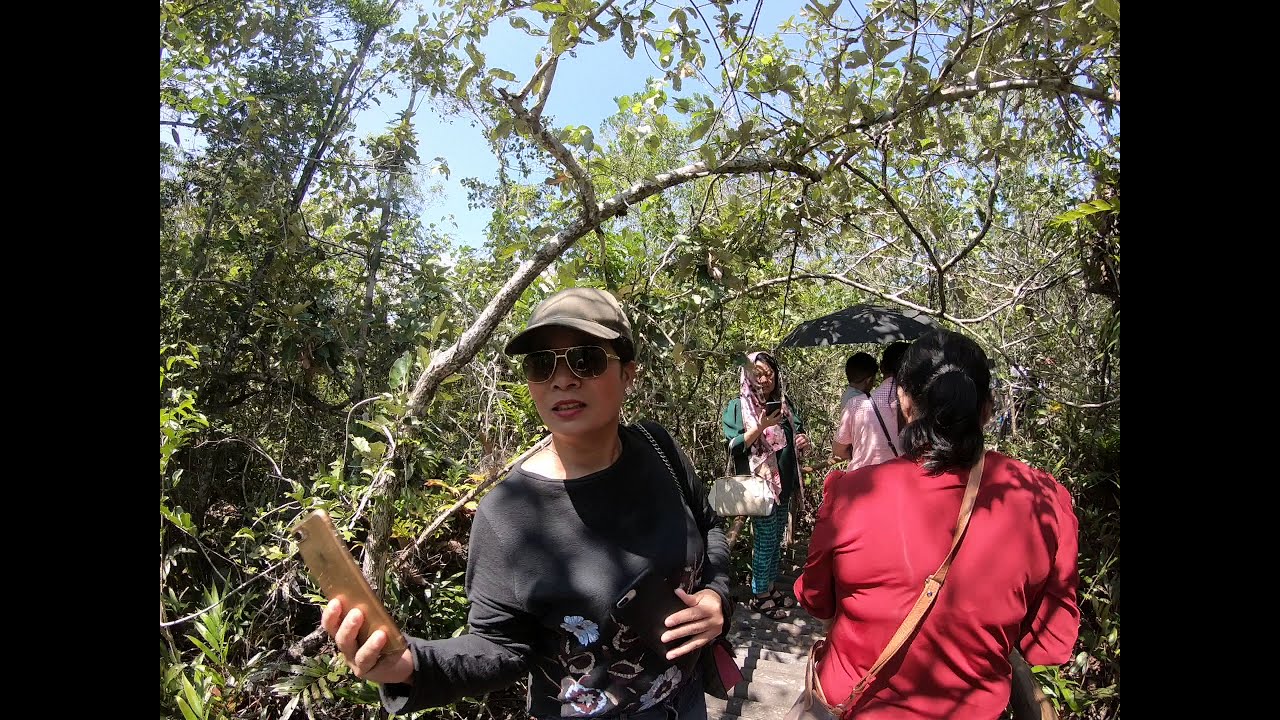On a bright, sunny day, a forest trail sprawls out under dappled sunlight filtering through the lush canopy. At the center of the image, a woman wearing a baseball cap, sunglasses, and a long-sleeved black shirt adorned with embossed flowers is holding a gold iPhone in her left hand, gazing off-camera. Her hair is tucked under her cap, and she has a purse slung over her shoulder. Behind her and slightly in the distance, another woman can be seen wearing a long teal dress and carrying a white handbag, with a scarf draped over her head. To the right, facing away, a woman in a red sweater with a brown leather strap across her shoulder walks away from the viewer, revealing a long line of people further down the trail. Among them, a figure clad in white uses an umbrella as a parasol. The vibrant blue sky peeks through the dense leaves, emphasizing the serene yet lively atmosphere of this picturesque forest trail.